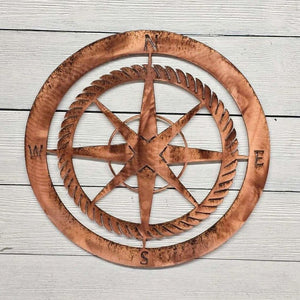The professionally staged, square full-color photograph features a wall-mounted decorative compass, possibly crafted from brass or copper. The background consists of vertical, gray painted wooden planks with visible black lines where the boards meet, suggesting an outdoor setting, though this is not entirely certain. 

The compass design is intricate and eye-catching: its outer ring, marked with the cardinal directions—N at the top, E to the right, S at the bottom, and W to the left—is engraved in black. Inside this ring is a toothed circle that resembles a saw blade. At the heart of the compass lies an eight-pointed star, extending in various directions, intersected by an "X" that signifies northeast, southeast, southwest, and northwest. Additional circles and shapes inside the compass further enhance its intricate design, making it a striking piece of wall art or a decorative product image.